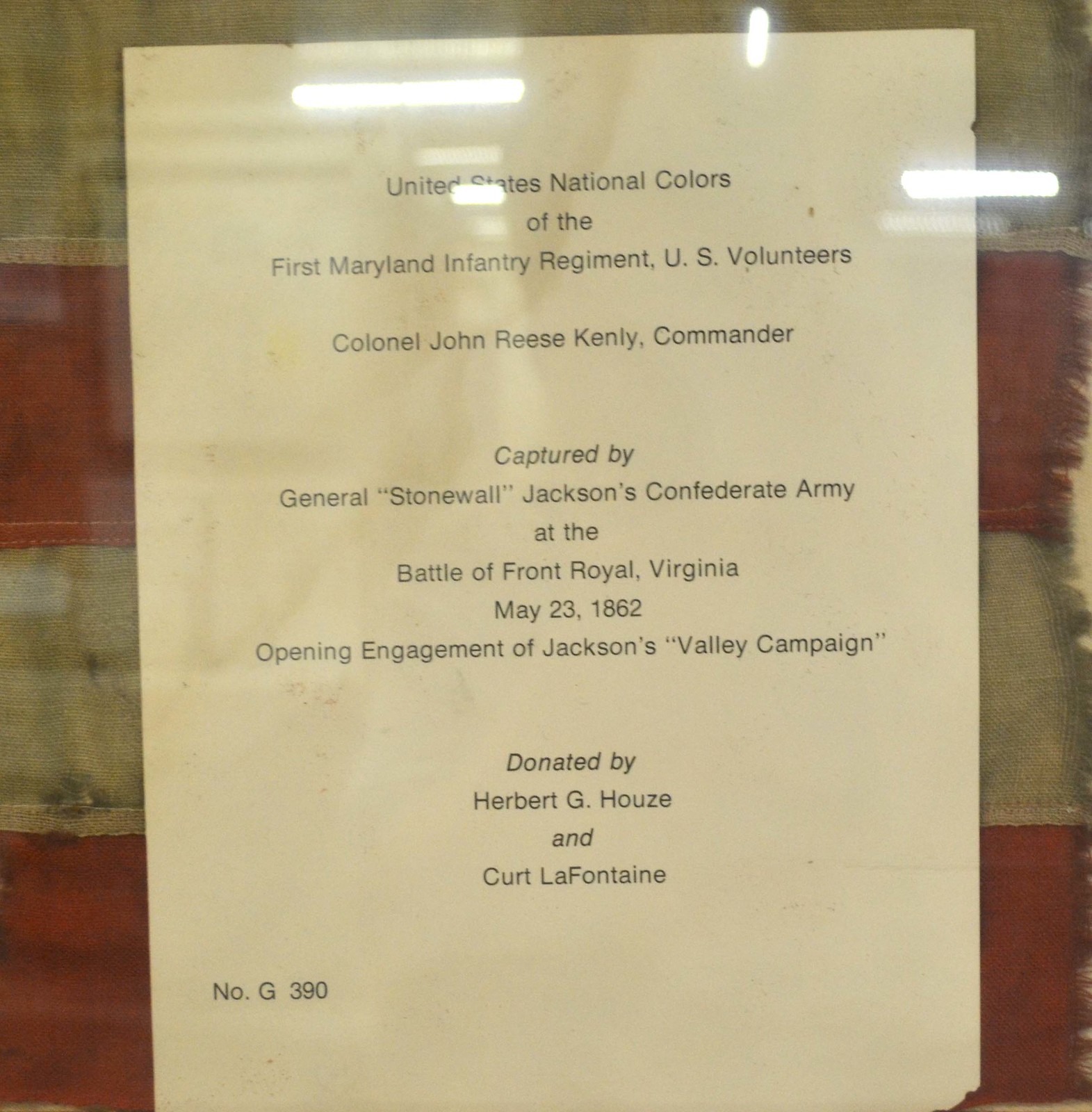This vertical rectangular photograph captures a piece of paper taped to a glass door, with light reflections making it somewhat difficult to read. The paper details the artifact in the background, describing it as the United States National Colors of the 1st Maryland Infantry Regiment, U.S. Volunteers, under Colonel John Reese Kenley. It further notes that this flag was captured by General Stonewall Jackson's Confederate Army during the Battle of Front Royal, Virginia, on May 23, 1862, marking an opening engagement of Jackson's Valley Campaign. The artifact was donated by Herbert G. Howes and Kurt LaFontaine, labeled with number G390. Behind the paper, partially visible, are red and white stripes suggesting the presence of the historic flag being described.